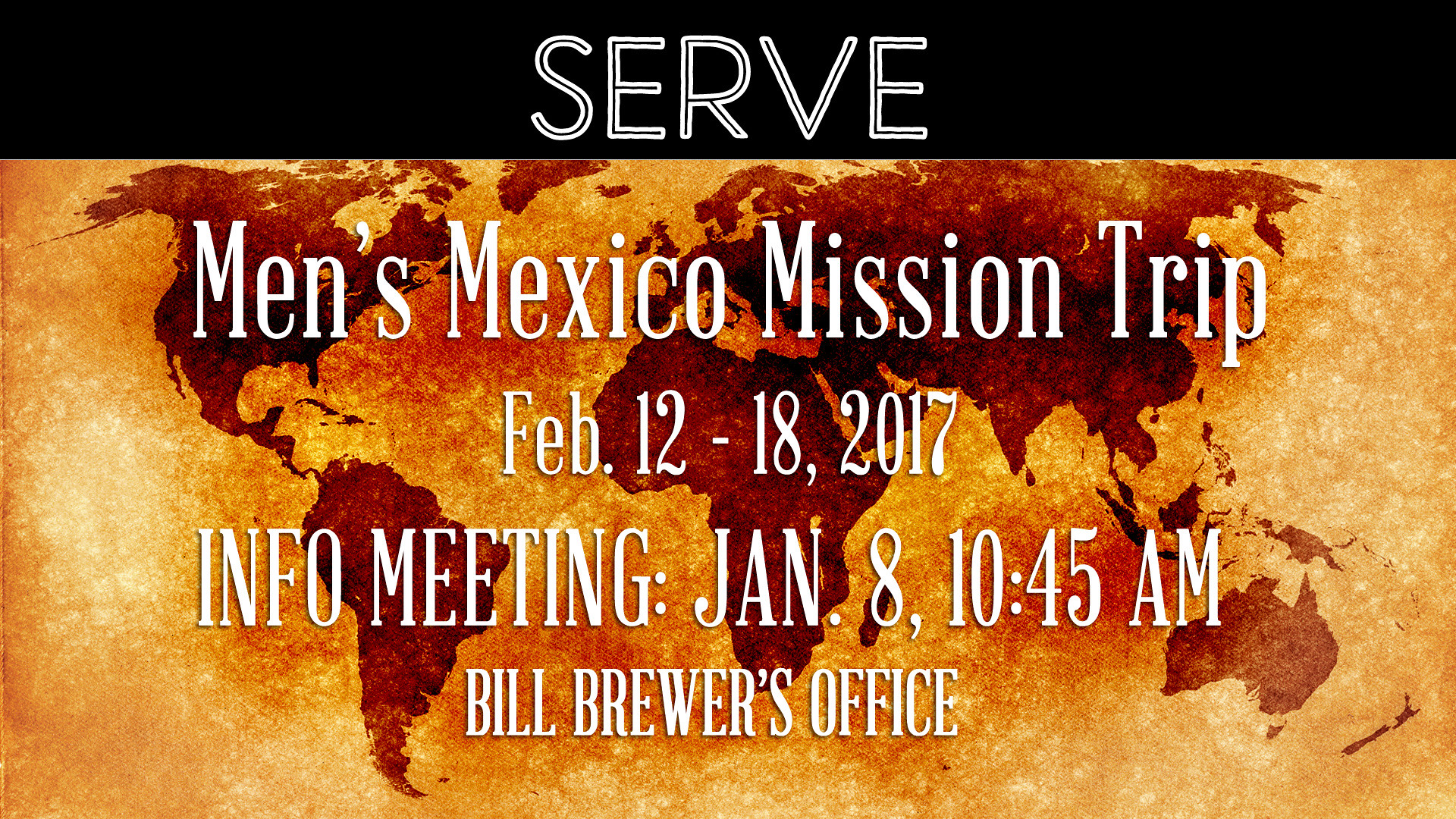This advertisement for a men's mission trip to Mexico features a captivating illustration and clear typography. The top portion of the image displays a black horizontal strip with the word "SERVE" boldly written in large white capital letters. Below this, a meticulously detailed antique-style watercolor and sepia-toned world map occupies the rest of the image. The continents are depicted in a dark reddish-brown while the oceans are rendered in lighter shades of reddish-browns, creating a warm yet engaging background. Superimposed on this map in tall, bold white font are four lines of text providing essential details: "Men’s Mexico Mission Trip," followed by the dates "February 12th through the 18th, 2017." Additional information about an info meeting scheduled for "January 8th, 10:45 a.m., Bill Brewer’s office" is also displayed, ensuring viewers have all the necessary details for participation.